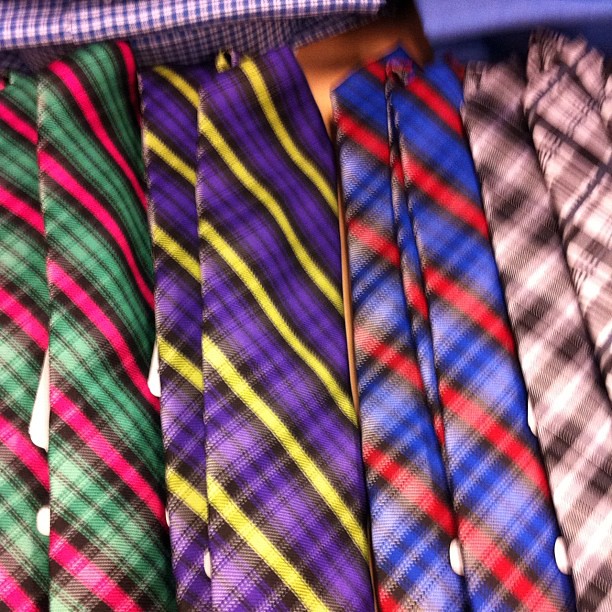This slightly blurry, square-shaped photograph appears to capture a neatly organized clothing display, possibly in a store. The background is a light brown, wooden surface, reminiscent of a table. Dominating the image are eight or nine ties meticulously arranged from left to right. Starting from the left, the first tie features green, black, and pink diagonal stripes. Next to it, the second tie displays purple, black, and yellow diagonal stripes, followed by a third tie with blue, black, and red stripes. The next tie on the right showcases a black and white criss-cross pattern. At the very top of the photograph, there are folded shirts: a white shirt with blue and red stripes on the top left and blue shirts located at the top right. An orange material appears to be partially visible behind the ties, enhancing the sense of a well-thought-out visual presentation typically found in retail displays.